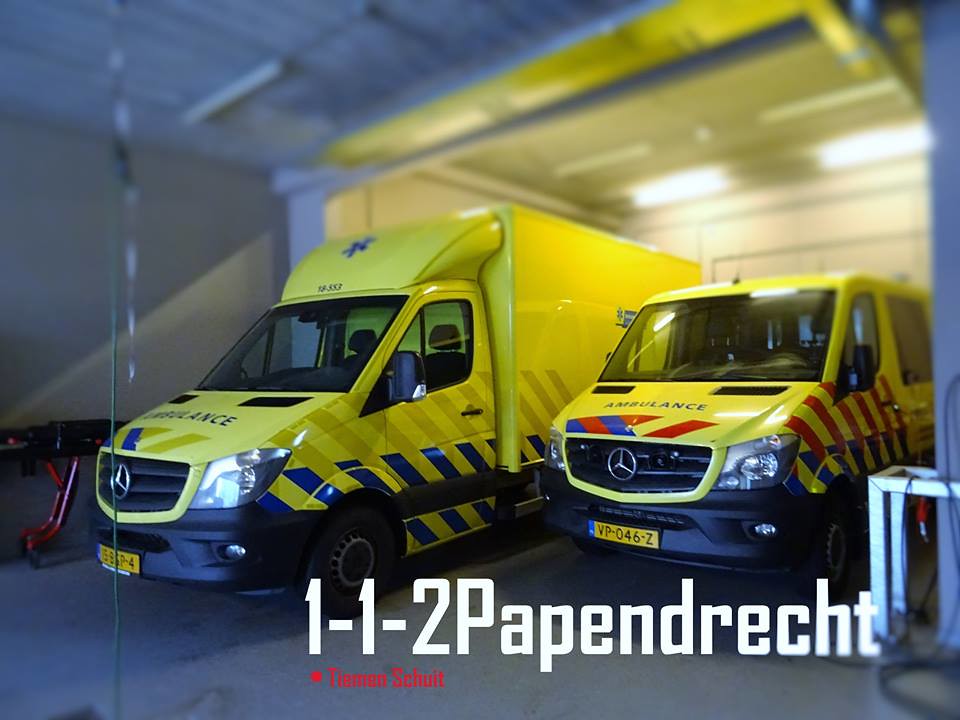The image features a large garage-like enclosure where two ambulances are parked side by side. The ambulance on the left is a larger, box truck-style vehicle with a yellow upper body and blue lower body, adorned with blue diagonal lines on the side. The smaller ambulance on the right is a passenger van, with a red upper body and blue lower body that includes vertical red stripes on the side. Both ambulances are Mercedes-Benz models. The van has additional markings reading "1-1-2 Papendrecht" on the bottom. The garage itself features a yellowish door at the bottom and a blue upper section, with the surrounding wall painted blue and white. This is evidently a designated parking area for the ambulances.